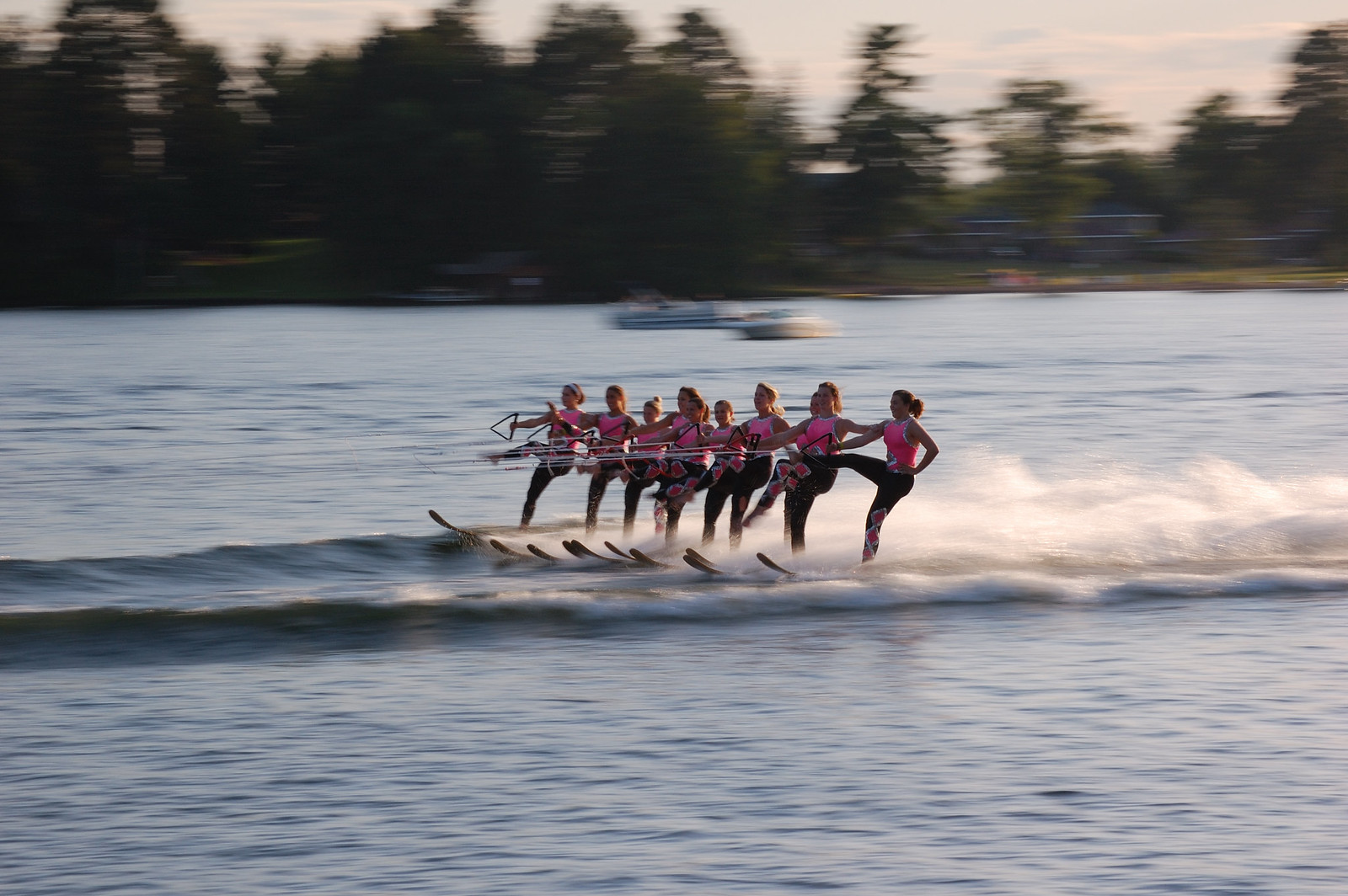This is a wide, horizontal, color photograph capturing a dynamic, synchronized water skiing performance on a large lake. The setting is outdoors during the daytime, with a slightly white sky and a backdrop of blurred green trees extending across the upper third of the frame. Just beyond the initial tree line, two slightly blurry speedboats dot the background, enhancing the sense of motion.

In the very center of the image, a striking formation of ten female water skiers, all in identical outfits, commands attention. They wear black leggings adorned with pink diamond accents on the calves and matching form-fitting, sleeveless pink tops. Each skier has her hair tied back and sports a distinct pose: one ski in the water, the right leg bent at a 90-degree angle, and left hand poised confidently on her hip while the right hand firmly grips the handle of a tow rope.

The water beneath them churns into a dramatic white wake, emphasizing their impressive coordination and balance. Although the boat pulling them isn't visible, the well-defined wake traces a direct line behind the skiers. The combination of synchronized motion, vivid colors, and blurred background captures the thrilling essence of this energetic water sport.